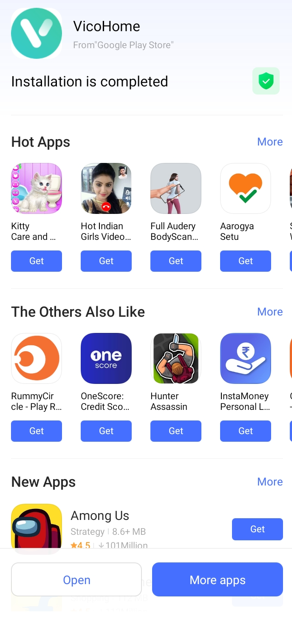The image displays the VicoHome interface, positioned prominently on the upper left-hand side. The brand name "VicoHome" merges "Vico" and "Home" together, with the 'V' in "Vico" and the 'H' in "Home" both capitalized. Adjacent to the brand name is a logo consisting of a green circle with a white 'V' in the center.

Beneath the title, a notification reads "Installation is completed." Following this message, the interface showcases three distinct sections: "Hot App," "Others Also Like," and "New Apps."

In the "Hot App" section, the featured apps listed are:
1. Kitty
2. Hot Indian Girls Video
3. Full Audrey Bodycam
4. AAROGYASETU.

The "Others Also Like" section suggests:
1. RummyCircle
2. OneScore: CreditScore
3. HunterAssassin
4. InstaMoneyPersonal.

Finally, in the "New Apps" section, the singular featured app is "Among Us," rated highly with 4.5 stars. A "Get" button is also visible to the right of this app listing.